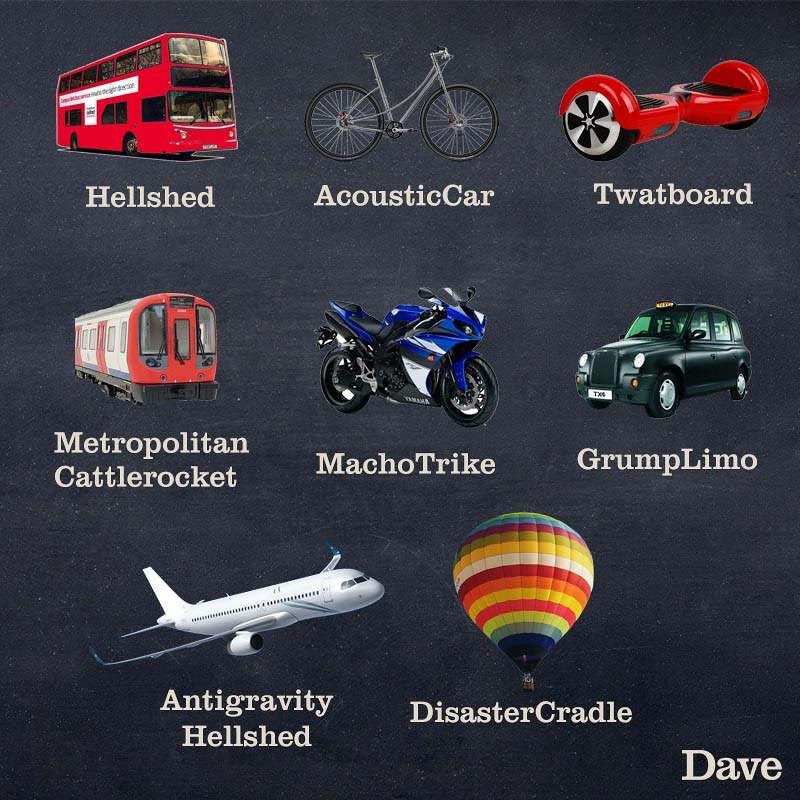The image in question shows a brochure with a dark, almost asphalt-colored background, featuring various modes of transportation arranged in a detailed layout. At the top left, there's a red double-decker bus labeled "Hell's Shed." Moving to the right, there's an image of a bicycle underneath which it says "Acoustic Car." Next to it, there's a two-wheel scooter labeled "Twad Board." In the bottom middle right section, there's an older car marked as "Grump Limo." At the center lies a blue motorcycle labeled "Macho Trike." Adjacent to it is a metro train named "Metropolitan Cattle Rocket." On the bottom left, a passenger airplane is labeled "Anti-Gravity Hell's Shed." Finally, to the right, there’s a multicolored hot air balloon named "Disaster Cradle." In the bottom right corner, the word "Dave" is clearly written in white letters. These images together illustrate a variety of transportation types, each whimsically titled, spread across the brochure in an organized manner with a total of eight displayed items formatted in two rows on top and a single row at the bottom.